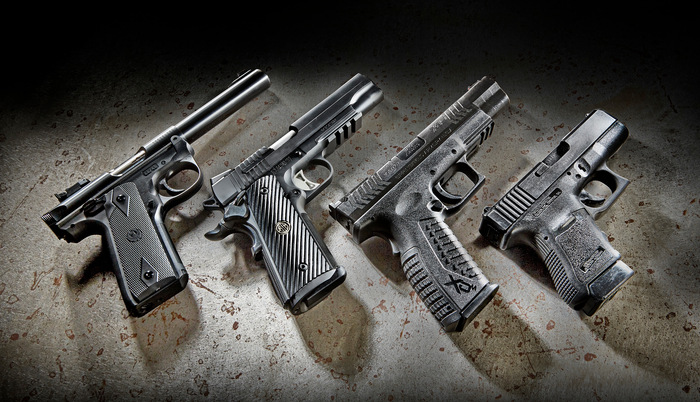The image showcases four black handguns placed in a precise arrangement, barrels all pointing to the top right corner against a bright, white background framed by a black border. Each firearm is distinctly visible due to the clear image quality and natural lighting. The guns are lined up from left to right, organized by their length and design features.

- The leftmost handgun is the longest with a smooth, thin barrel and a lightly textured handle.
- The second handgun is slightly shorter, featuring a thicker barrel and a handle textured with diagonal ridges. It also has a lighter gray trigger mechanism.
- The third handgun is almost the same length as the second but slightly shorter. It has a thick barrel and a handle that is partially textured and partially smooth, bearing the inscription "XJM" or "XO".
- The rightmost handgun is the shortest and thickest. Its handle is textured only on the back, with the top part of the handle being smooth.

Overall, the handguns are positioned in a clean, bright setting, on a terrazzo-like surface with some colored flecks visible on the background.